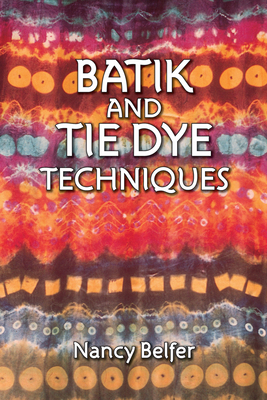The image depicts the cover of a book or manual titled "Batik and Tie-Dye Techniques," authored by Nancy Belfer, whose name appears at the bottom of the cover. The title is prominently centered on the cover, written in white text outlined in black. The background showcases an array of intricate Batik and tie-dye designs, featuring various shapes such as squares, circles, and smaller circles. The vibrant and diverse color palette includes shades of purple, white, orange, magenta, blue, gray, beige, deep purple, reds, browns, and golds. The patterns and colors are expertly arranged, with no bleeding into one another, creating a striking and cohesive visual effect that evokes the dynamic and fluid qualities of a lava lamp. The colors transition smoothly across the cover, adding to its visual appeal. Overall, the cover is a beautiful and detailed representation of the artistic techniques described within the book.